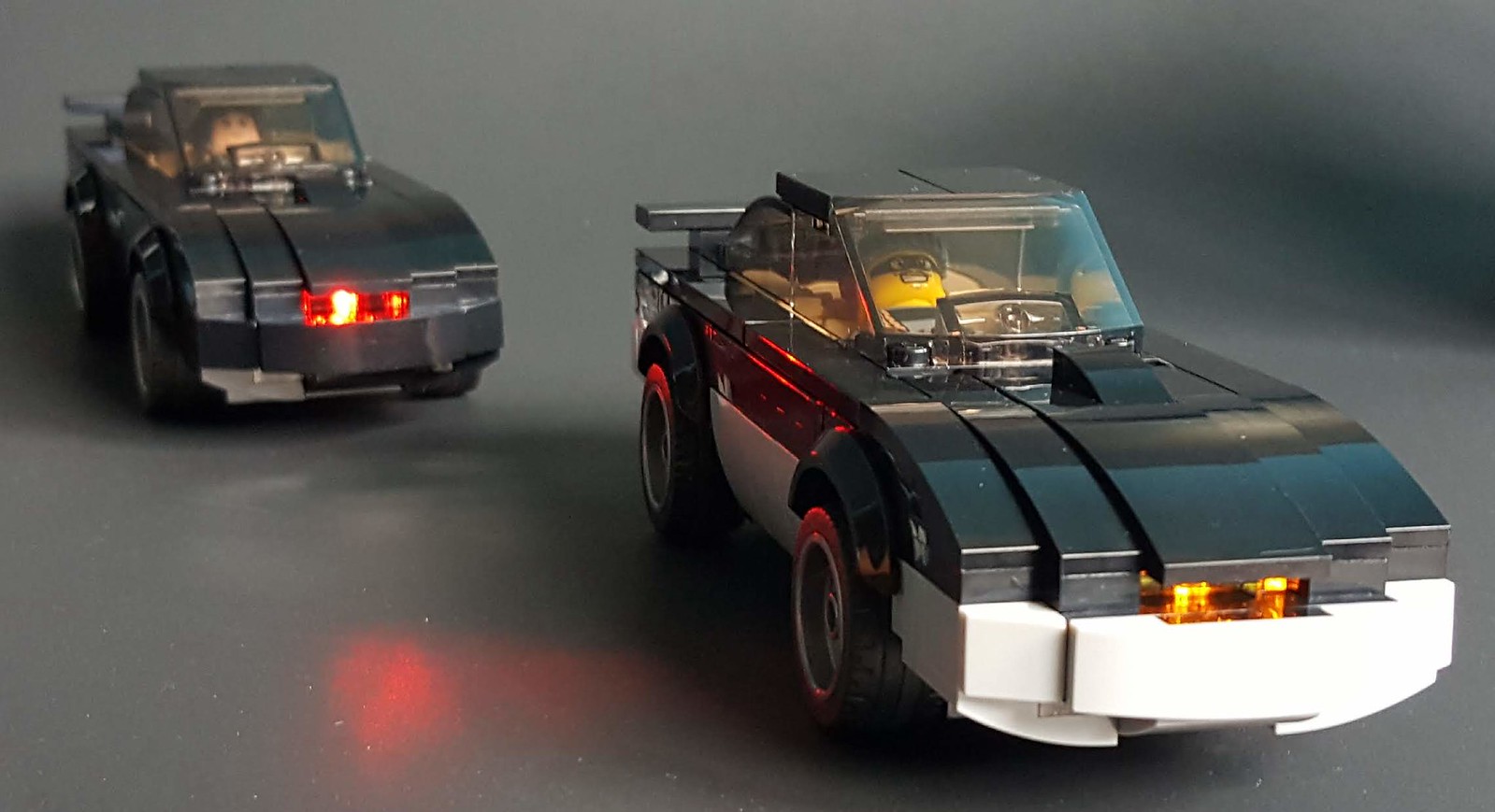This indoor photograph captures a close-up, angled view of two sophisticated Lego race cars positioned on a gray tabletop. One car, predominantly black with a white lower half and yellow front lights, is in the foreground and in sharp focus. This car features a grimacing Lego figure, styled as a robber with a black mask and a striped shirt, seated in the driver’s seat. The second car, slightly out of focus in the background, mirrors the design of the first but is entirely black with red front lights. Its driver is another Lego figure with peach-colored skin, lacking the robber’s distinctive mask and attire. The red lights on this car cast a reflection on the tabletop, highlighting the attention to detail in this meticulously staged scene.